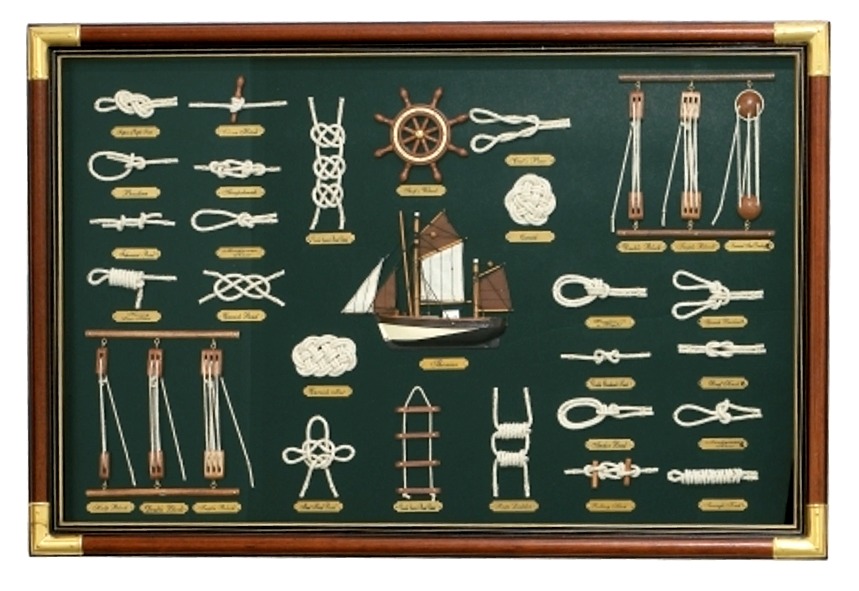This landscape-oriented photograph showcases a framed display of various nautical rope ties, meticulously presented as a piece of artwork. The frame is crafted from attractive redwood and is accentuated with brass or gold corners and a complementary gold and black inner border. The background of the display is a deep, forest green color, enhancing the maritime theme.

Central to the display is a small model of an old sailing ship featuring white and brown sails, accompanied above by a wooden-handled nautical steering wheel that radiates like a clock. Around the ship model, the artwork features an array of approximately 20 to 25 different sailing knots, each piece of white rope carefully tied and labeled with golden plaques indicating the name and type of knot.

Additionally, the display includes examples of pulley systems, with components like levers and wooden pulleys that are used for raising and lowering sails on ships. These pulleys are positioned on both the bottom left and top right corners of the artwork, enhancing the educational and aesthetic value of the exhibit. The detailed presentation combines elements of historical sailing techniques and nautical craftsmanship in a beautifully framed and informative piece.